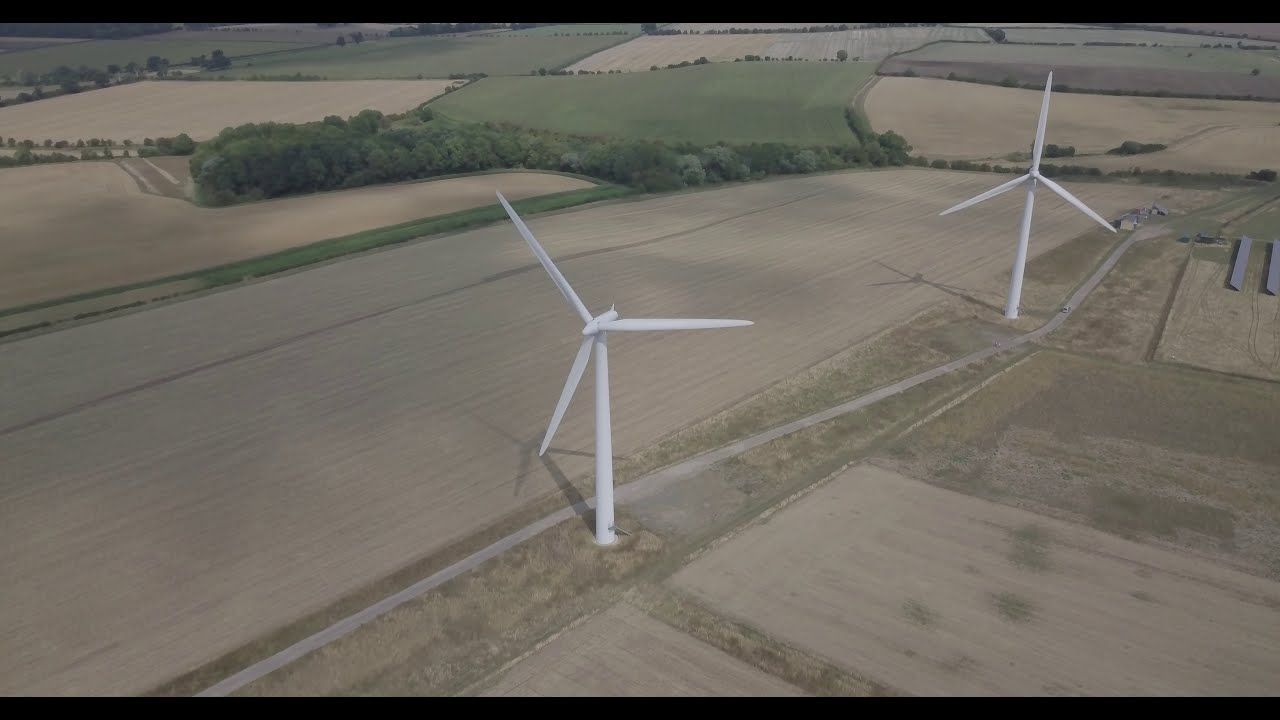The image features a peaceful, rural landscape dominated by two modern wind turbines used for electricity generation. Both turbines are white with three arms each, situated amidst fields that appear to have been harvested for the winter, giving them a brownish-gray hue. There are contrasting patches of green fields, with a notable green section to the north of the image. The turbines are arranged with one centrally located and the other positioned towards the top right. A dirt road runs from the bottom of the image, winding towards the top right, flanked by the harvested fields. To the west, there is a shaded area of green trees and lush green fields, giving the scene a vibrant yet serene feel. Additionally, there is a car near the turbines in the far north, and some buildings can be observed on the right side of the image, accentuating the rural setting. Overall, the scene captures the harmony between technological advancement and the natural countryside.